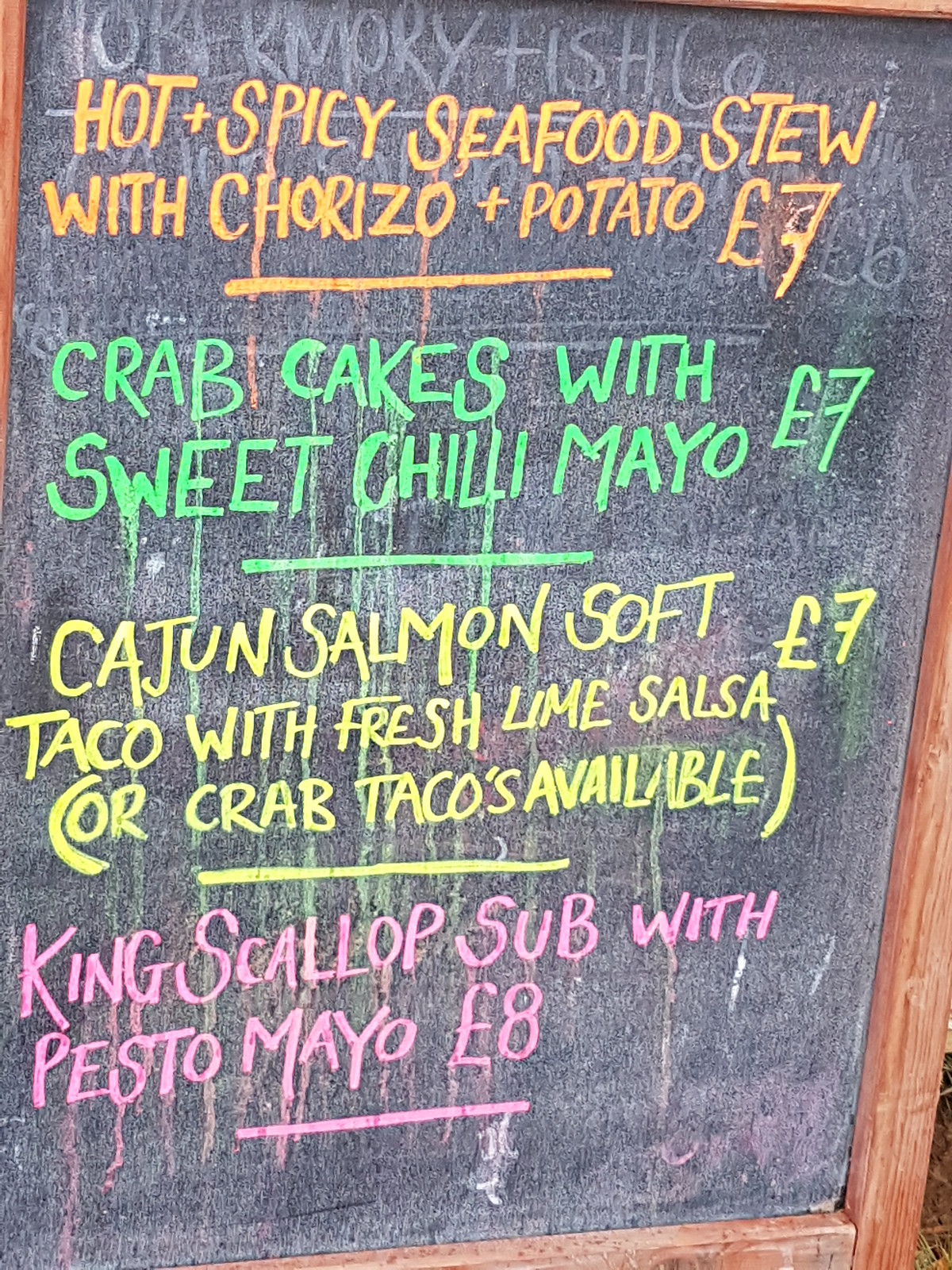In this portrait-style outdoor photograph, a vintage wooden frame encases a black chalkboard stand-up sign, slightly askew and placed in a bright mid-day setting. The chalkboard, possibly belonging to a restaurant named Toramori Fish Co., prominently features a specials menu written in vibrant chalk colors, albeit with visible chalk dust and ghost words from previous entries.

The menu is divided into four sections, each in different colors:
1. **Orange:** "Hot & Spicy Seafood Stew with Chorizo & Potato" - priced at £7.
2. **Green:** "Crab Cakes with Sweet Chili Mayo" - priced at £7.
3. **Yellow:** "Cajun Salmon Soft Taco with Fresh Lime Salsa or Crab Tacos Available" - priced at £7.
4. **Pink/Purple:** "King Scallop Sub with Pesto Mayo" - priced at £8.

The image captures the rustic charm and frequent updates exhibited by the layered chalk writings, encapsulating a vivid snapshot of the restaurant's enticing seafood offerings.